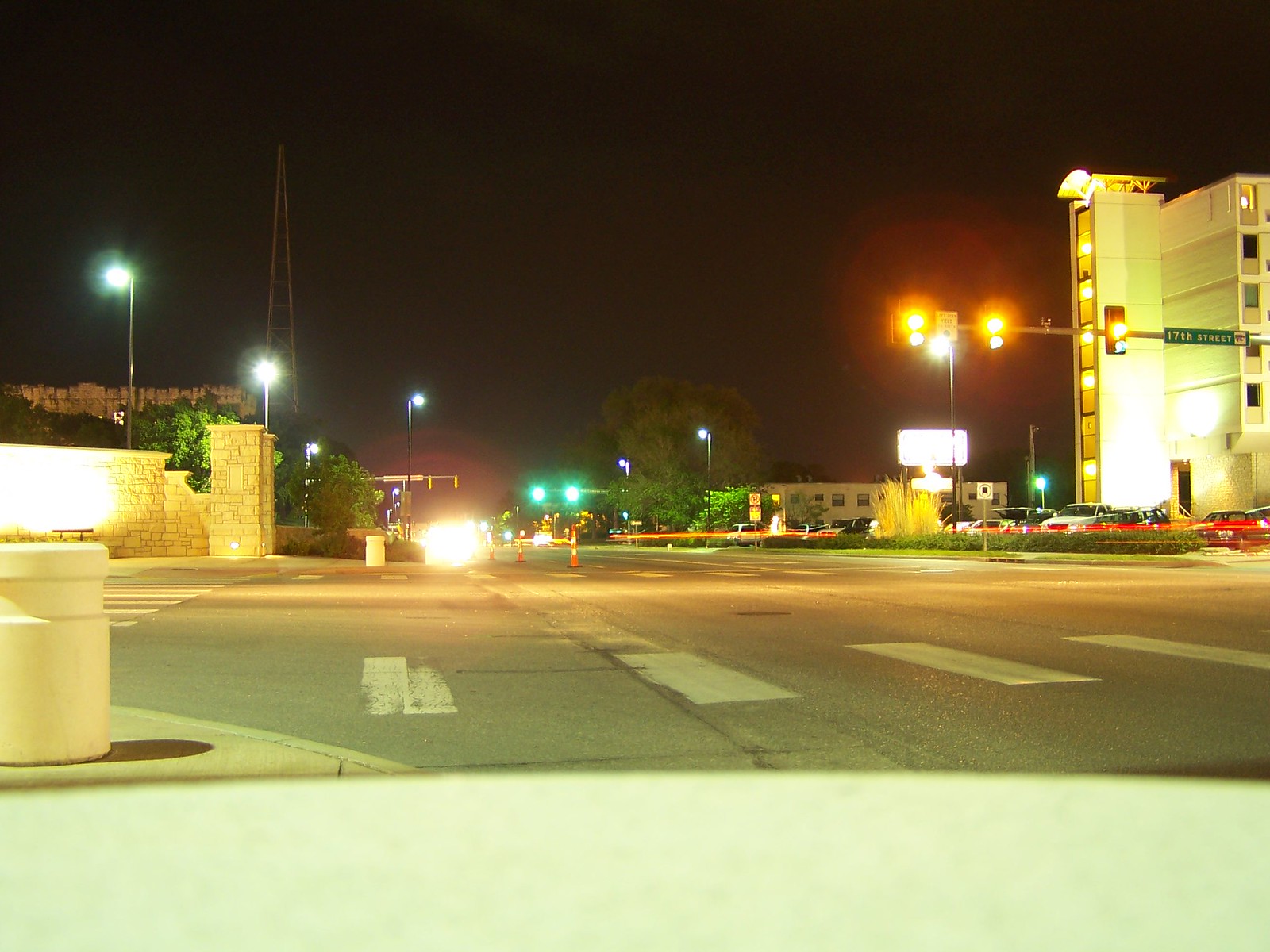In the evening, an empty intersection is illuminated by street lights and a green traffic signal. To the right, a building with an indistinct structure stands, casting shadows on its surroundings. A street sign with yellow lights glows softly nearby. The left side of the scene features a brick wall, possibly marking the entrance to a hotel, adding a touch of sophistication to the urban landscape. A billboard looms in the background, barely visible in the dim light. Ahead, the crosswalk stretches across the street, undisturbed by pedestrians. In the middle-left distance, headlights from an approaching car break the stillness, yet it remains far away. The day appears dry, with no signs of recent rain, contributing to the calm atmosphere.